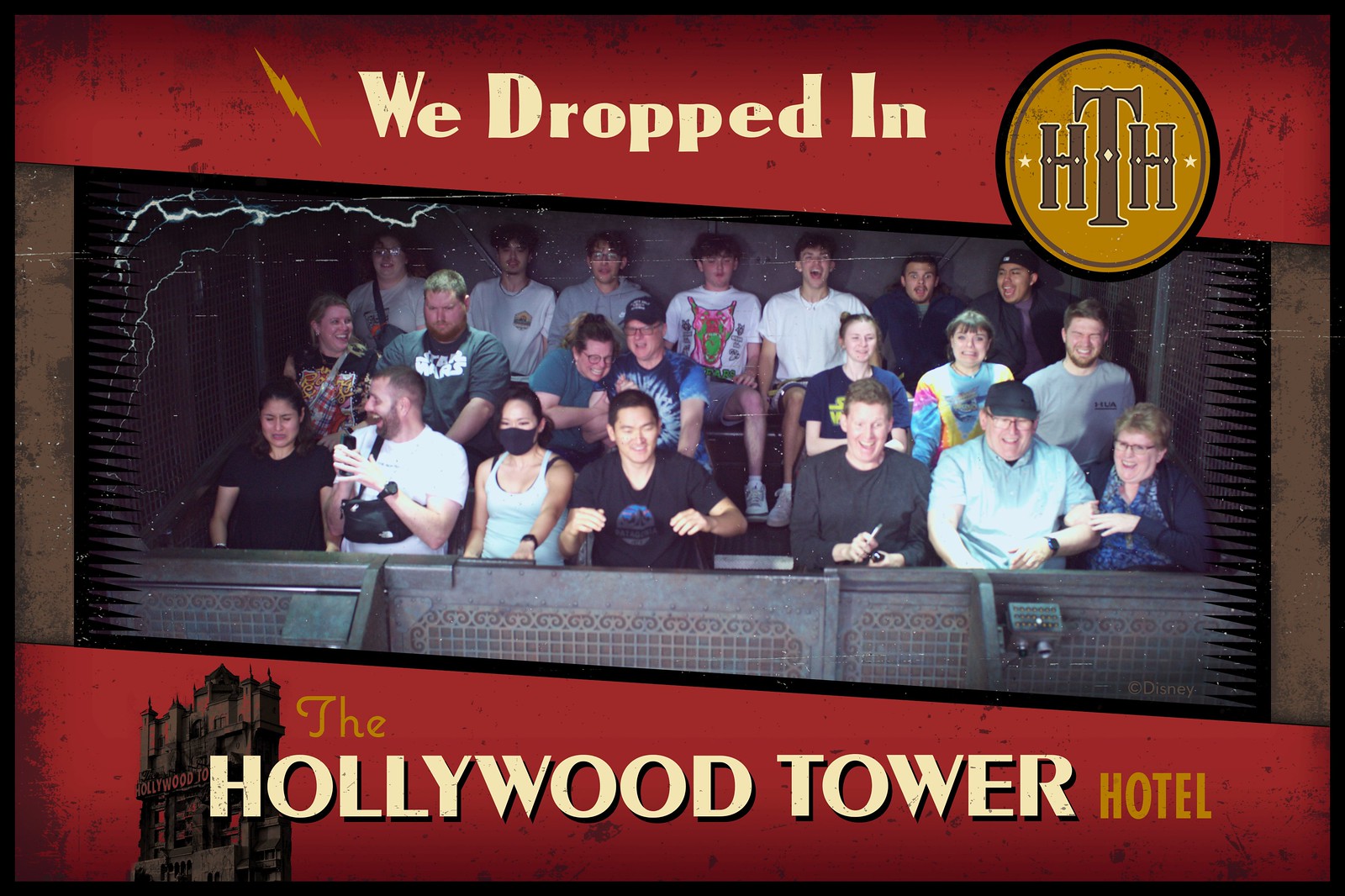In the photo, there is a group of people experiencing a thrilling ride, likely at a theme park attraction called the Hollywood Tower Hotel. The text framing the top and bottom of the photo reads, "We dropped in, the Hollywood Tower Hotel," suggesting this image was taken during the ride and later purchased as a keepsake. The scene resembles an elevator filled with passengers, arranged in three rows—approximately eight people on the top row, seven in the middle, and six on the bottom. Everyone is facing the camera, with emotions ranging from excitement and happiness to fear. One notable detail is a woman in the front row on the left with her eyes tightly shut, looking terrified, while the man next to her in a white or gray shirt laughs. The spooky theme is further emphasized by a lightning bolt effect added across the top of the image. The overall color scheme includes shades of red, orange, white, and brown, enhancing the vintage, eerie aesthetic of the Hollywood Tower Hotel ride experience.